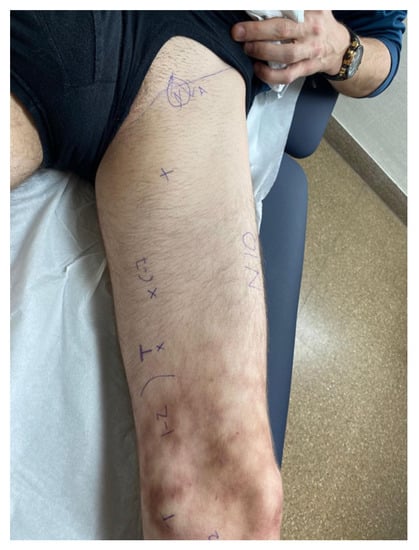This image depicts a white male patient sitting on an exam table in a doctor's office, with his shorts and underwear pulled up to expose his leg from the groin to just below the knee. His leg, which is thin and has sparse dark hair, shows multiple bruises and does not appear healthy. It is extensively marked with blue ballpoint pen, featuring various symbols and letters, including "N-A" at the groin, an "X" at mid-thigh, "1 - 2" near the knee, and other annotations like "T - X," "+," and "NIO." These markings suggest upcoming surgery. The background includes a gray-cushioned exam table covered with a white sheet, the patient's arm with a black and gold wristwatch, and part of the hospital room with a speckled beige floor and gray molding at the base of a white wall. Another person, possibly a doctor, is faintly visible in the background.